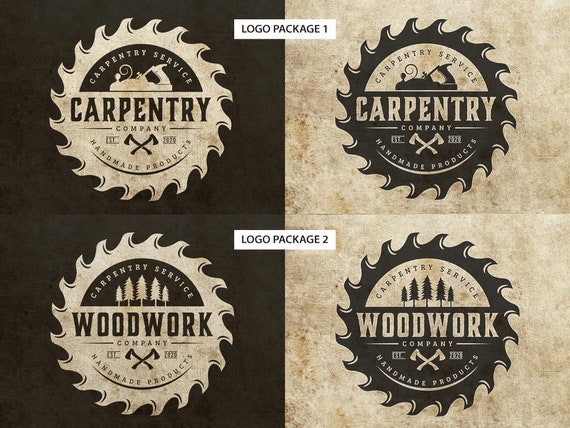This image features four distinct logos, grouped into two packages for a carpentry company. The top half of the image is labeled "Logo Package 1" and contains two logos, one on the left and one on the right. Both logos display in a square format with a saw wheel design. The left logo has a dark brown background featuring a tan saw wheel with crossed axes forming an X. The text "Carpentry Company, Carpentry Service, Handmade Products" is inscribed in black. The right logo is a color-inverted version of the left, with a tan background and dark brown saw wheel and text.

The lower half is labeled "Logo Package 2" and includes another set of two logos. Similar to the top, the left logo has a dark brown background with a tan saw wheel. However, this time the text reads "Woodwork Company, Handmade Products" and features a row of trees at the top. The right logo again inverts the colors, displaying a tan background, dark brown saw wheel, text, and the tree design at the top. The alternating color schemes between the packages provide a visual variety while maintaining consistency in the design elements.